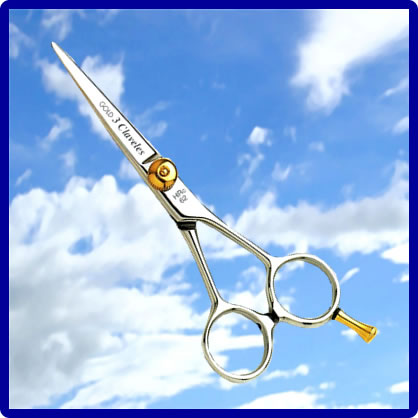This image features a compact, stainless steel pair of scissors laying diagonally against a vivid blue sky with scattered white clouds. The scissors extend from the upper left corner to the lower right corner of the image. A distinctive gold screw secures the center pivot, while a small gold prong juts out from one of the finger holes. The glossy, silver blades bear the inscription "3 Clavicles" in black text. The realistic sky background is framed by a darker blue border, creating a sharp contrast that makes the scissors appear as though they're floating in mid-air. These shears are likely designed for precise tasks such as sewing, trimming fabric, or haircutting.